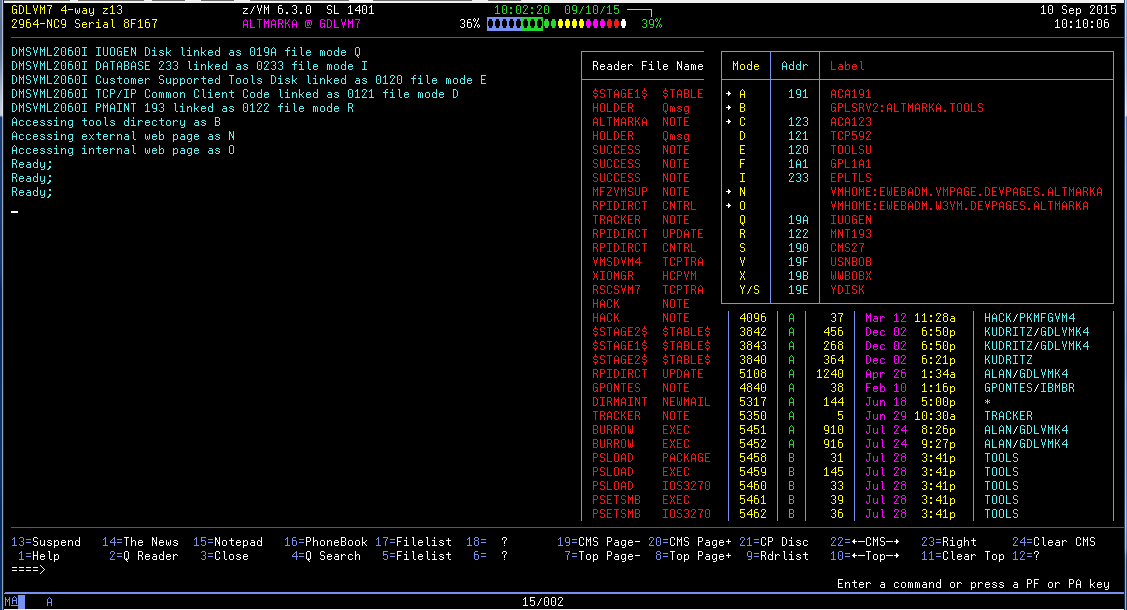The image is a screenshot of a vintage computer console, reminiscent of systems from the 1980s or 1990s. It features a simple interface with a black background and text displayed in a variety of colors, including red, yellow, cyan, green, and purple. There are no modern graphical elements or windows present, only text.

On the left side of the screen, there are several console commands such as "accessing tools directory as B" and "accessing internal web page as O," followed by a "ready" prompt, indicating that this section is where the user inputs commands to interact with the computer.

The right side of the screen displays text in red, listing what appear to be file names like "tracker," "hack," and "stage_2." Each file name is accompanied by additional information such as different numeric values and descriptors, which likely represent file sizes and dates marking when the files were last accessed or updated. This detailed arrangement provides a snapshot of the computer's directory and its contents, offering insight into the commands and files accessed by the user.